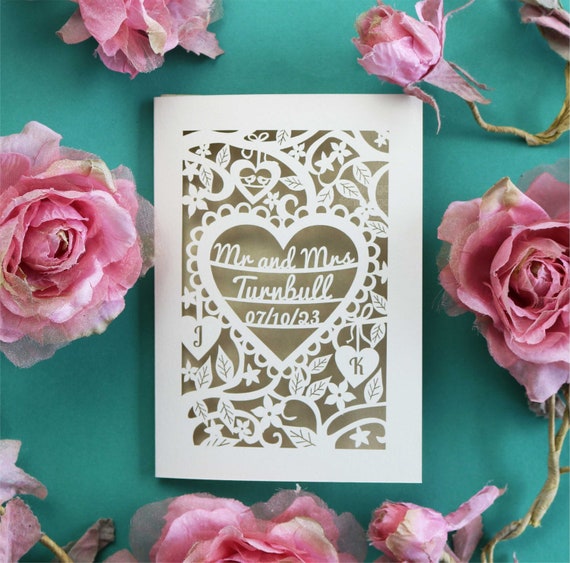In this meticulously staged photograph, a stunning wedding invitation card is showcased front and center on a light aqua-green surface. The card itself is predominantly white, featuring finely detailed paper cut-outs and delicate gold embellishments. It reads "Mr. and Mrs. Turnbull, 7-10-23," with the letters "J" on the left and "K" on the right. Surrounding this beautiful card are an array of artificial roses in varying shades of rose pink, complemented by pale blue-green and light purple-green accents, as well as brownish-green stems. The careful arrangement of these elements highlights the creative and professional design of the invitation, suggesting that the photograph is intended for an online marketplace or a catalog.